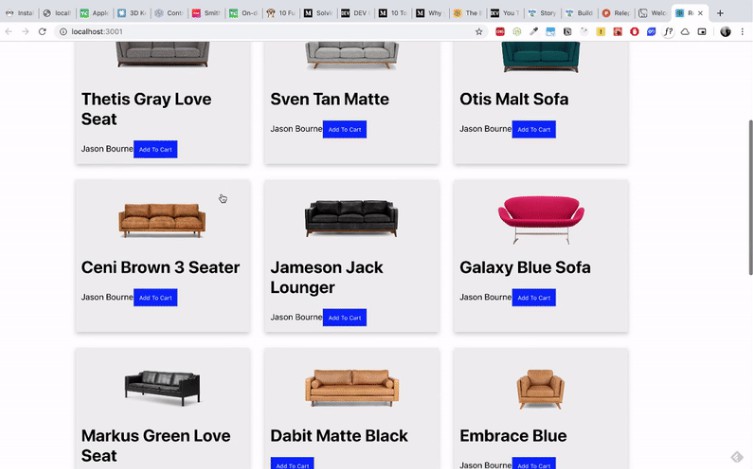This detailed caption provides an elaborate description of an image captured from a webpage displaying a variety of couches, each housed within a gray box. Each gray box contains a couch with its respective details and purchasing options:

At the top, we see:
1. A gray three-seater couch labeled "Thetis Gray Love Seat," accompanied by the name "Jason Bourne" and a blue "Add to Cart" button. 
2. Beside the gray couch is another couch named "Sven Tan Mate," spelled as 'S-B-E-N.' This also includes "Jason Bourne" and a blue "Add to Cart" button.
3. Moving forward, a green couch is featured, titled "Otis Malt Sofa," which also has a blue "Add to Cart" button.

Going further down:
4. There's an orangish-brown couch referred to as "Sunny Brown Three Seater," alongside its blue "Add to Cart" button.
5. Centrally located among these listings is a "Jameson Jack Lounger," which also includes a blue "Add to Cart" button.
6. Next, there's the "Galaxy Blue Sofa."

In another section:
7. It showcases a "Marcus Green Love Seat."
8. Following that is "Debit Mate Black."
9. Lastly, an "Embrace Blue."

Each of these couches is individually presented with clear labeling, and each features a convenient blue "Add to Cart" button for easy purchasing.